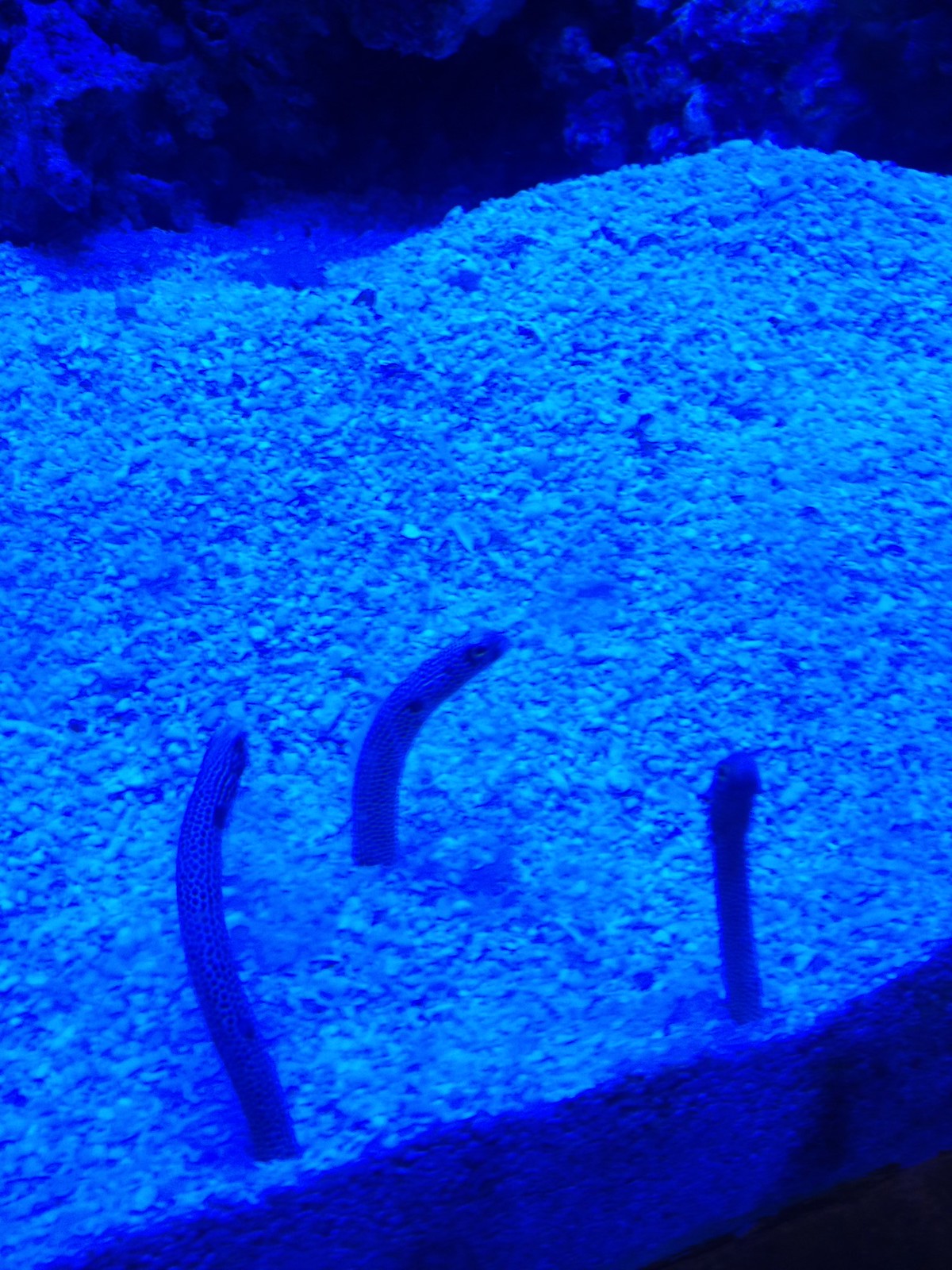This underwater photograph, taken in various shades of blue, features a prominent rocky surface in the center. The rock is smooth and highlighted by mineralization or crystals that give it a shinier appearance. Three worm-like creatures, dark and textured, emerge from the rock, with one standing almost upright and the others curving slightly. The background reveals darker, blurred rocky formations, adding depth to the image. The sandy surface beneath the rock, in hues of purple and white, contrasts against the darker backdrop, creating a striking composition reminiscent of an aquarium scene.